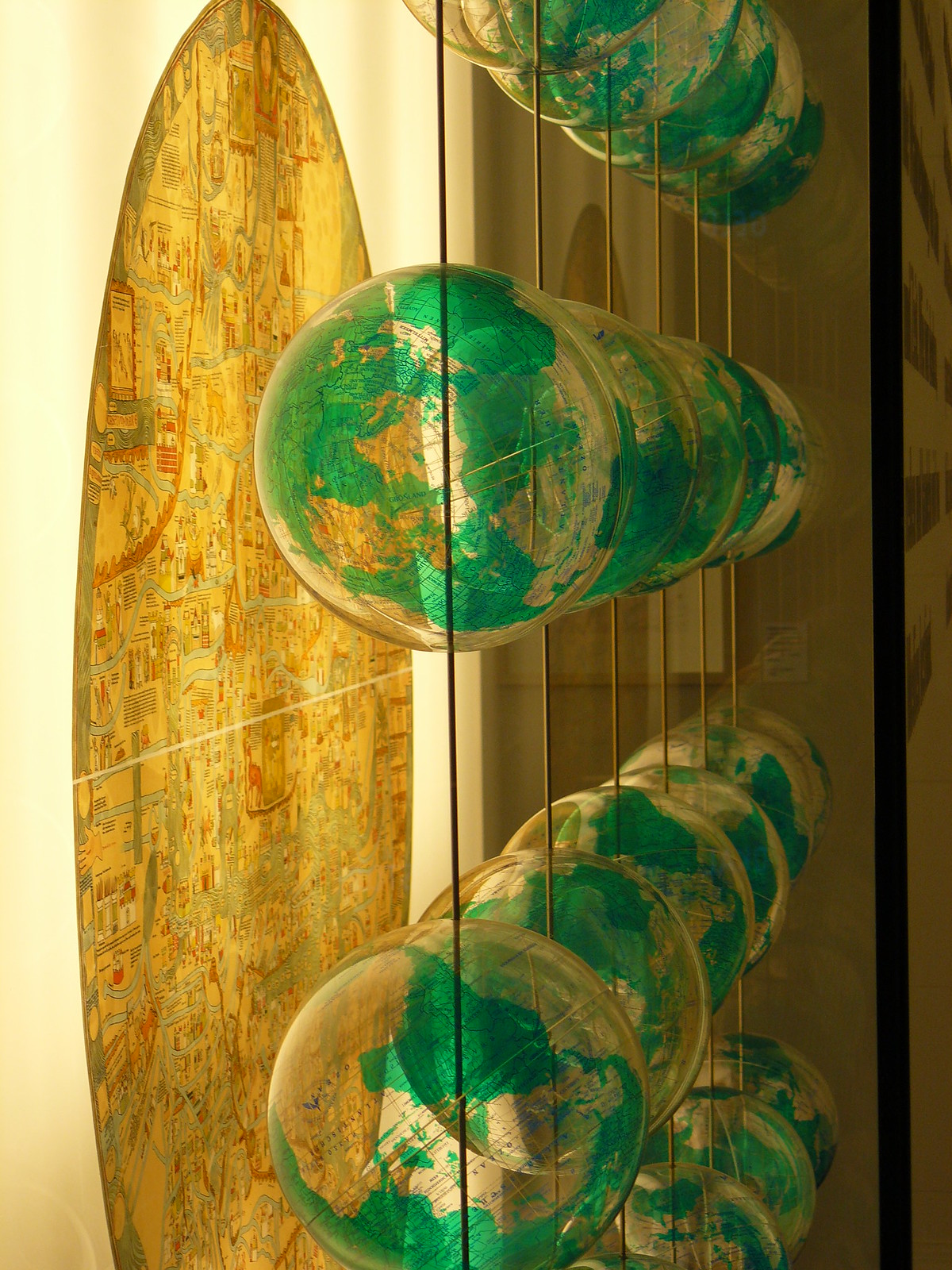The photograph, presented in color and portrait orientation, captures an intriguing room interior featuring two distinct elements. On the left, a long, oval-shaped wooden board, reminiscent of an aged surfboard, leans against a beige surface. Adorned with yellow and orange markings, it gives the appearance of a map, possibly depicting a town, city, or state. To the right, a series of clear glass globes, distinguished by bluish-green water and golden land masses, are displayed on tiered glass shelves. Each globe is supported by a thin metal rod running vertically through the arrangement. The overall composition juxtaposes the aged wooden board against the modern and transparent glass globes, creating a visually captivating contrast within the room.